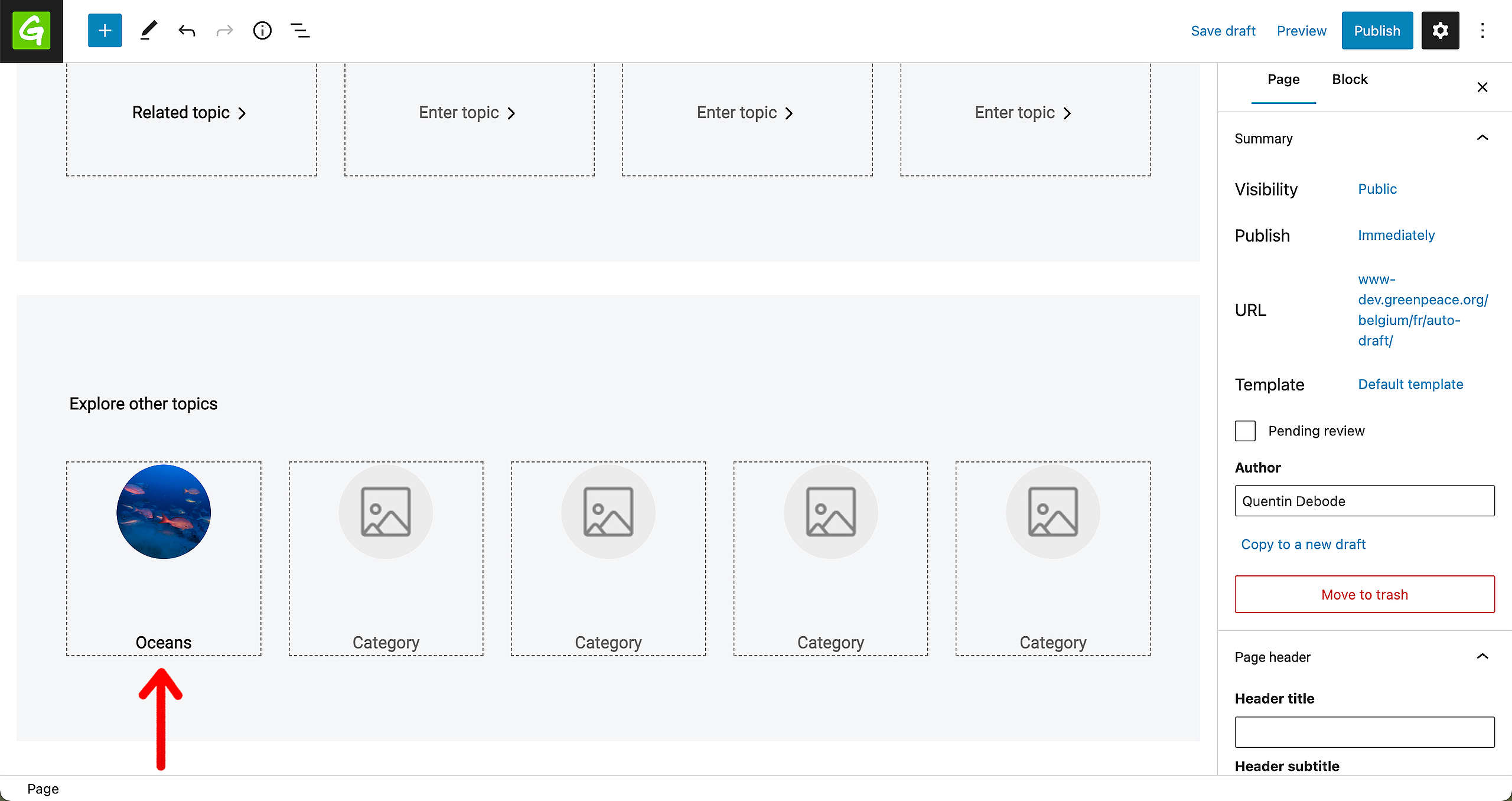In this intricate image, a digital console panel is displayed prominently, showcasing an array of text and functional elements. At the top, various navigation buttons such as "Save Drafts," "Preview," and "Publish" are clearly visible, along with a settings menu icon. Below these, there is a section prompting users to "Enter Topic" in three distinct input fields, labeled as the first, second, and third boxes, respectively.

To the right of these fields, there is a segment titled "Explore Other Topics," with "Oceans" listed as one of the featured categories. Associated with this, a sizable red arrow directs attention downward towards the "Oceans" box. Following this, the image displays four individual boxes, each labeled with different "Categories."

Further to the right, additional options and settings are detailed, including text references to "Visibility," which is set to "Public," and an option to "Publish Immediately." There are also selections related to "Templates," with "Default Templates" mentioned. The overall layout is bordered with various interface elements that frame the content effectively, drawing the user’s focus to the interactive and navigational aspects of the console panel.